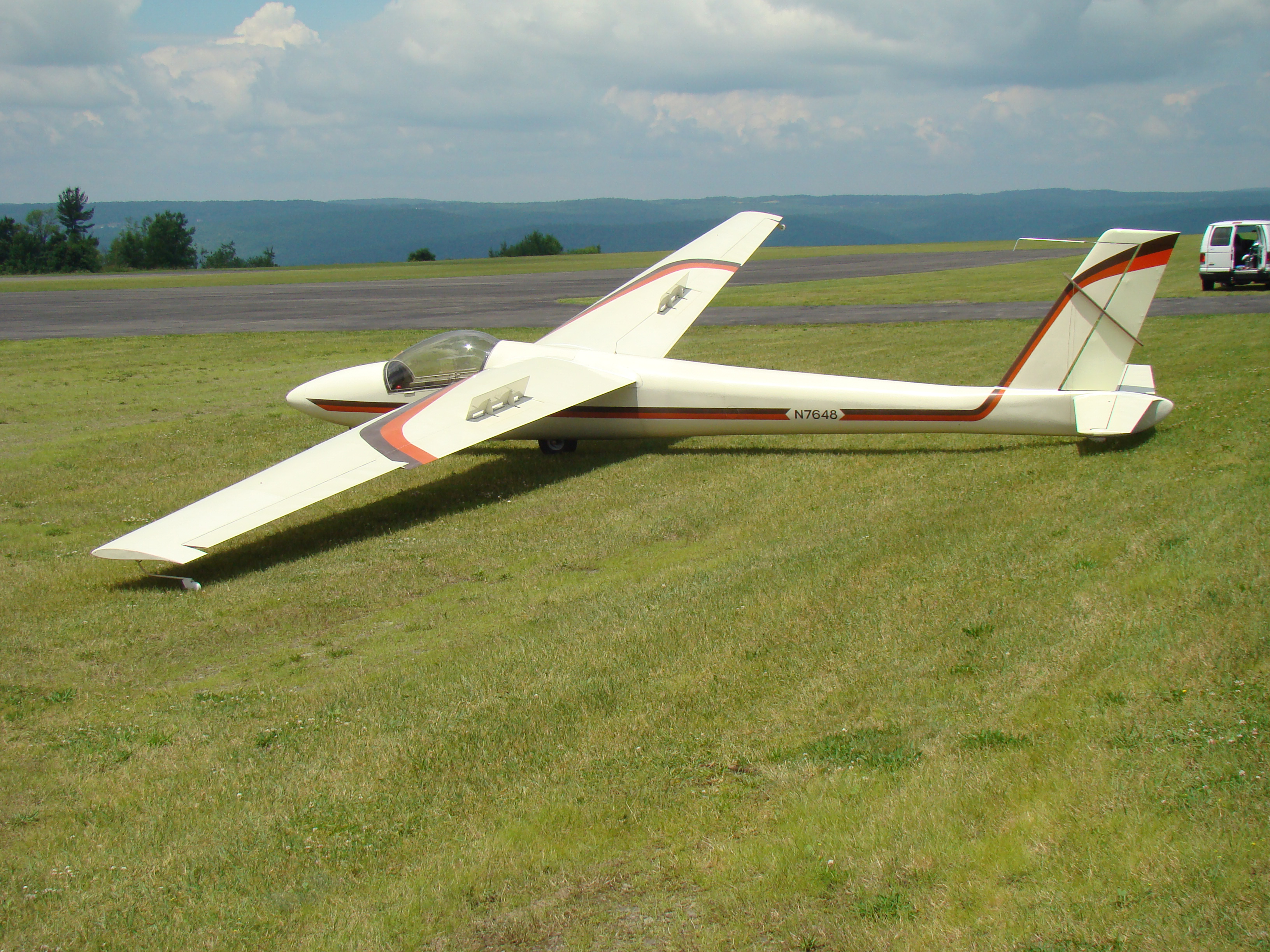In this image, we see a sleek, single-seat glider resting on a green grassy field adjacent to a paved runway. The glider is white with distinct red and black stripes. These stripes run from the nose cone along the fuselage, extending up to and across the top of the tail fin, and are also visible atop the wings. The glider is recognized by its clear, domed cockpit characteristic of engineless aircraft designed for gliding. The vehicle stands on its left wing, which touches the ground, while the right wing remains elevated. 

To the right of the frame, a white van with its back door open is positioned partly on the runway. The background boasts a picturesque scene with a mixture of blue, cloudy skies above, and a landscape featuring a row of green trees leading to distant, light-blue mountains. The backdrop includes a notable drop-off, revealing a large body of water, possibly a lake or the ocean, blending harmoniously with the idyllic elements of nature surrounding the runway and glider. The aircraft's identifying code "N7648" is marked within the stripe on its body.